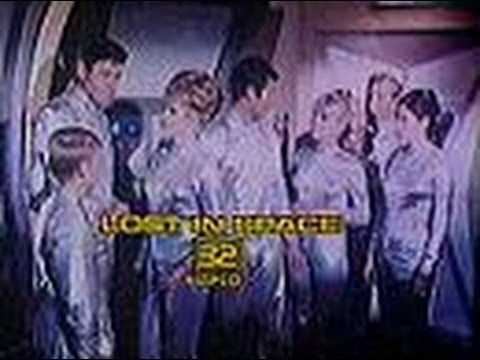The photo captures a group of seven individuals—three women, three men, and a boy—inside a cabin, all styled in the fashion of the 1970s. The image possesses a light purple color tone and features a notably pixelated and blurry quality. At the center of the photo is a yellow caption that reads "Lost in Space 32," although the text is somewhat difficult to read due to the image's overall blur.

Arranged in two main groups, the first group on the left consists of a dark-haired man standing next to a strawberry-blond boy and a woman with reddish hair. This trio is engaged, looking inward at each other. A second group is positioned to the right, featuring a central man flanked by two women and another man behind them. The central woman has blonde hair tied in a ponytail, while the other woman has brown hair also styled in a ponytail. All individuals are clothed in full-body silver outfits, enhancing the photo's distinctive period vibe. Each person's gaze and positioning create a dynamic scene focused around the central man, lending a sense of narrative intrigue to the image.